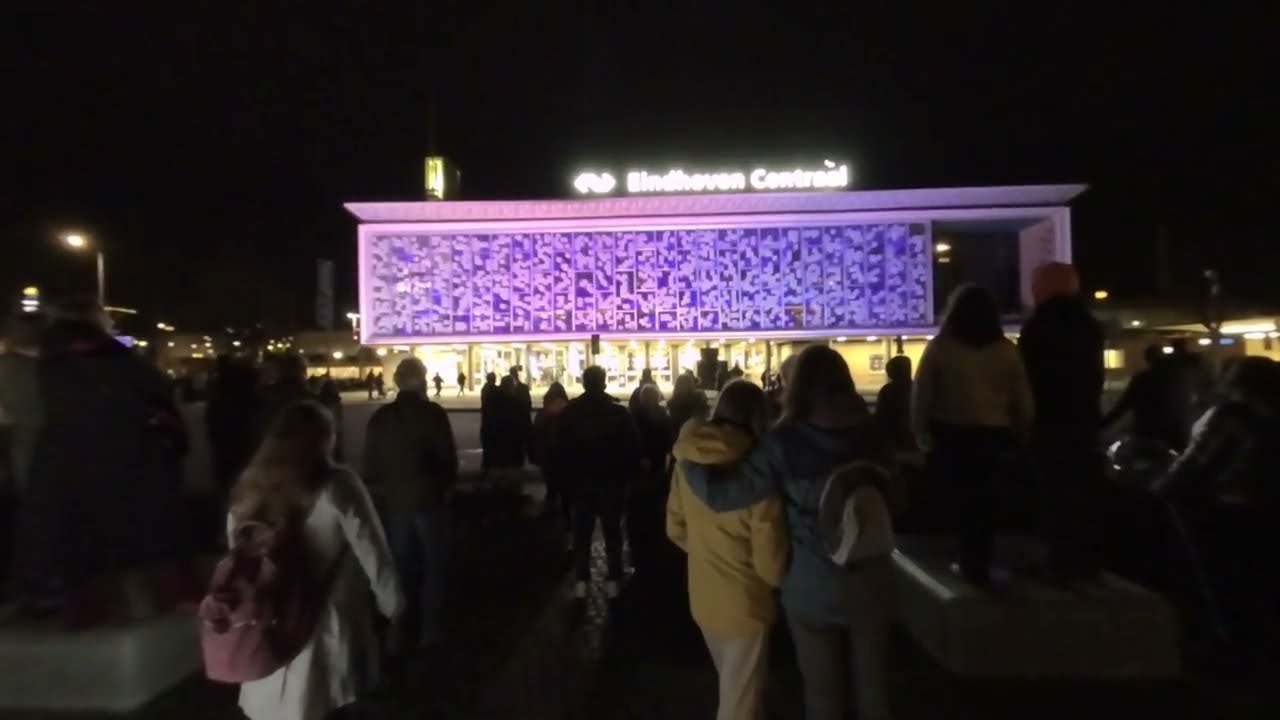This nighttime outdoor photograph captures a bustling scene where a crowd of people is walking towards a modern, brightly lit building in the background. Most of the individuals in the frame are seen from behind, emphasizing their focus on the building ahead. In the foreground, there is a notable detail of two women embracing in the right center of the image; one is wearing a yellow top with white pants while the other is dressed in dark pants and a dark jacket. Another woman to their left has on a white shirt and a pink backpack. 

The large building they are heading towards features a flat, rectangular, and contemporary design accented with numerous windows. The lower part of the building is illuminated with yellow lights, and through these windows, the interior is visible. Above this, the façade transitions into intricate patterns with blue and purplish hues, topped by a prominent band of purple near the roofline. Dominating the rooftop in bright white, lit-up letters is the sign "Eindhoven Centraal." The sky above is dark, enhancing the contrast of the illuminated structure against the night.